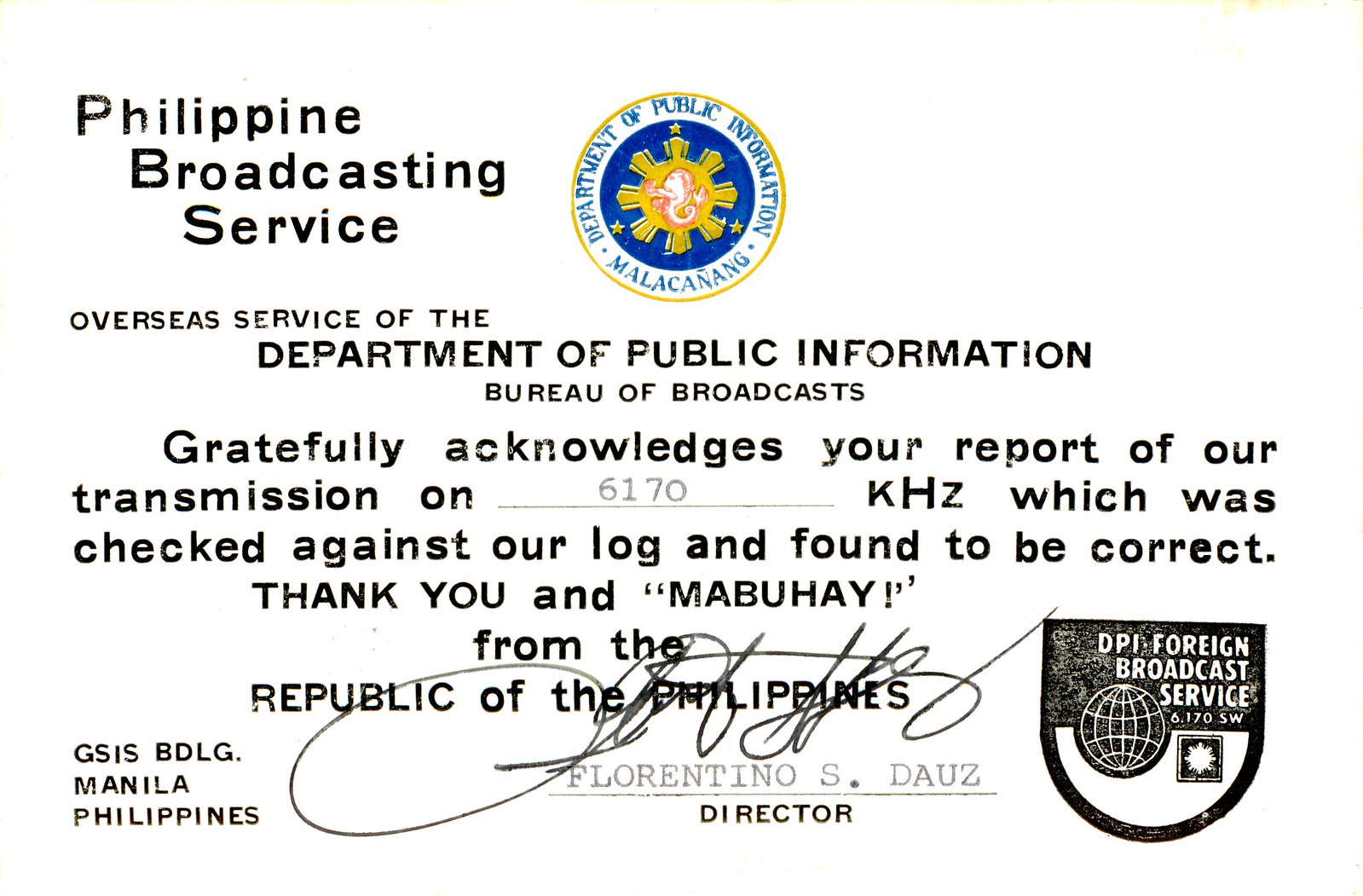This is an image of a bulletin, predominantly in black and white, with official details and a distinctive blue and gold seal at the top. The seal prominently features the words "Department of Public Information, Malacanang," accompanied by a yellow sun and three stars, with a detailed blue and red central design, possibly depicting a sea creature. The text in the top left corner categorizes the issuer as the "Philippine Broadcasting Service," a part of the "Overseas Service of the Department of Public Information, Bureau of Broadcasts."

The main body of the text acknowledges the receipt and verification of a transmission report on the frequency 6170 kHz, stating, “Gratefully acknowledges your report of our transmission on 6170 kHz, which was checked against our log and found to be correct. Thank you and Mabuhay from the Republic of the Philippines.” This acknowledgment comes with the signed name "Florentino S. Dauz," labeled as the Director.

The bottom left corner of the bulletin mentions the location as "GSIS Building, Manila, Philippines," while the bottom right corner highlights an emblem with the inscription "DPI, Foreign Broadcast Service," featuring a black and white globe design.